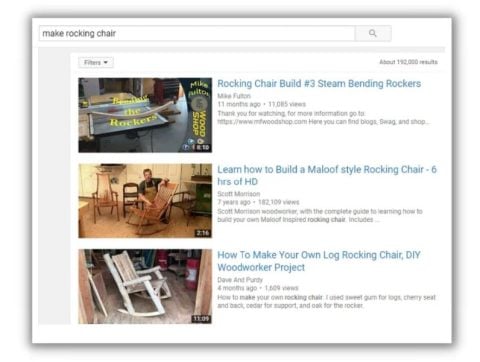The image features a white background with a search interface at its top center. The search bar displays the query "make rocking chair," and to the right of it, there is a small gray button with a magnifying glass icon indicating search functionality. Directly below this, a section with a gray background is predominantly filled by a large white box. In the top left corner of this section, there is a gray filter dropdown button. To its right, the text "About 192,000 results" is displayed.

Underneath this, a horizontal line separates the results area, where three options are presented:

1. The first option includes a thumbnail image of a table with the bottom of a rocking chair on it. The right side of this thumbnail reads "Rocking Chair Build Number Three: Steam Bending Rockers" by Mike Futon. This video was posted 11 months ago and has garnered 11,885 views. The caption includes a note of appreciation and directs viewers to visit Mike's website, https://www.mfwoodshop.com, for more information, blogs, merchandise, and shopping options.

2. The second option showcases an image of a man with light skin and dark hair sitting in a room next to a rocking chair. Two additional chairs are placed to his right. The accompanying description on the right reads "Learn How to Build a Maloof Style Rocking Chair," a 6-hour HD instructional video by Scott Morrison from 7 years ago with 182,109 views. Scott Morrison, a woodworker, offers a comprehensive guide on how to construct a Maloof-inspired rocking chair.

3. The third option displays a wooden rocking chair. The right side description states "How to Make Your Own Rocking Chair: DIY Woodworker Project" by Dave and Purdy, posted 4 months ago with 1,609 views. The tutorial details using materials like sweet gum for logs, cherry for the seal, back setter for support, and oak for the rocker.

This detailed caption captures the essence and specifics of the image, making it easily understandable and descriptive.